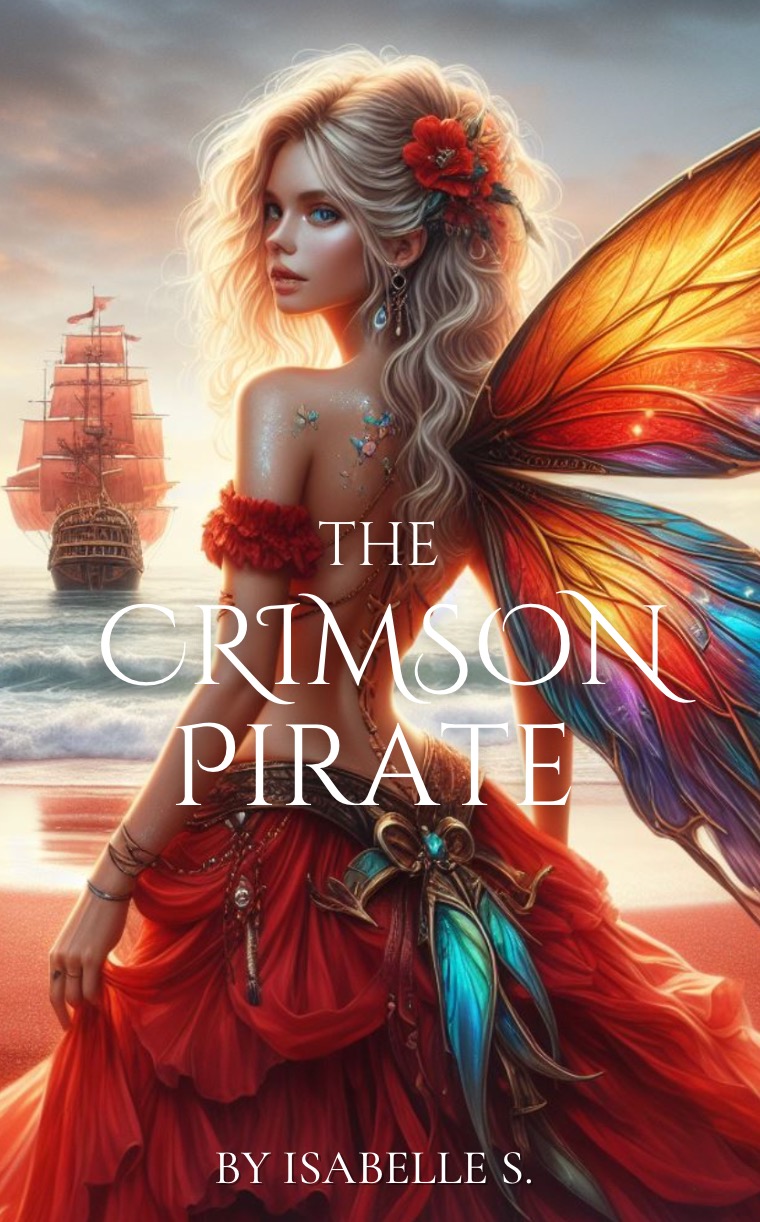The image depicts a digitally created book cover for "The Crimson Pirate" by Isabelle S. At the forefront stands a petite, beautiful young woman with long, wavy blonde hair adorned with red flowers. She has enchanting blue eyes and wears blue and black drop earrings. Her off-shoulder top, revealing her waist, is complemented by a floaty red garter skirt with a metallic blue-green bow accessory. Glitter embellishes her shoulders and neck, enhancing her magical aura. She possesses majestic, multicolored butterfly-like wings in shades of yellow, red, blue, and purple. 

In the background, a ship with light red sails sails gracefully towards her, reflecting a serene sky in the wet sand. The overall scene has a fantastical and ethereal quality, suggesting a blend of adventure and magic that perfectly matches the story's title. The title "The Crimson Pirate" is displayed in white, with the author's name, Isabelle S., noted beneath it.